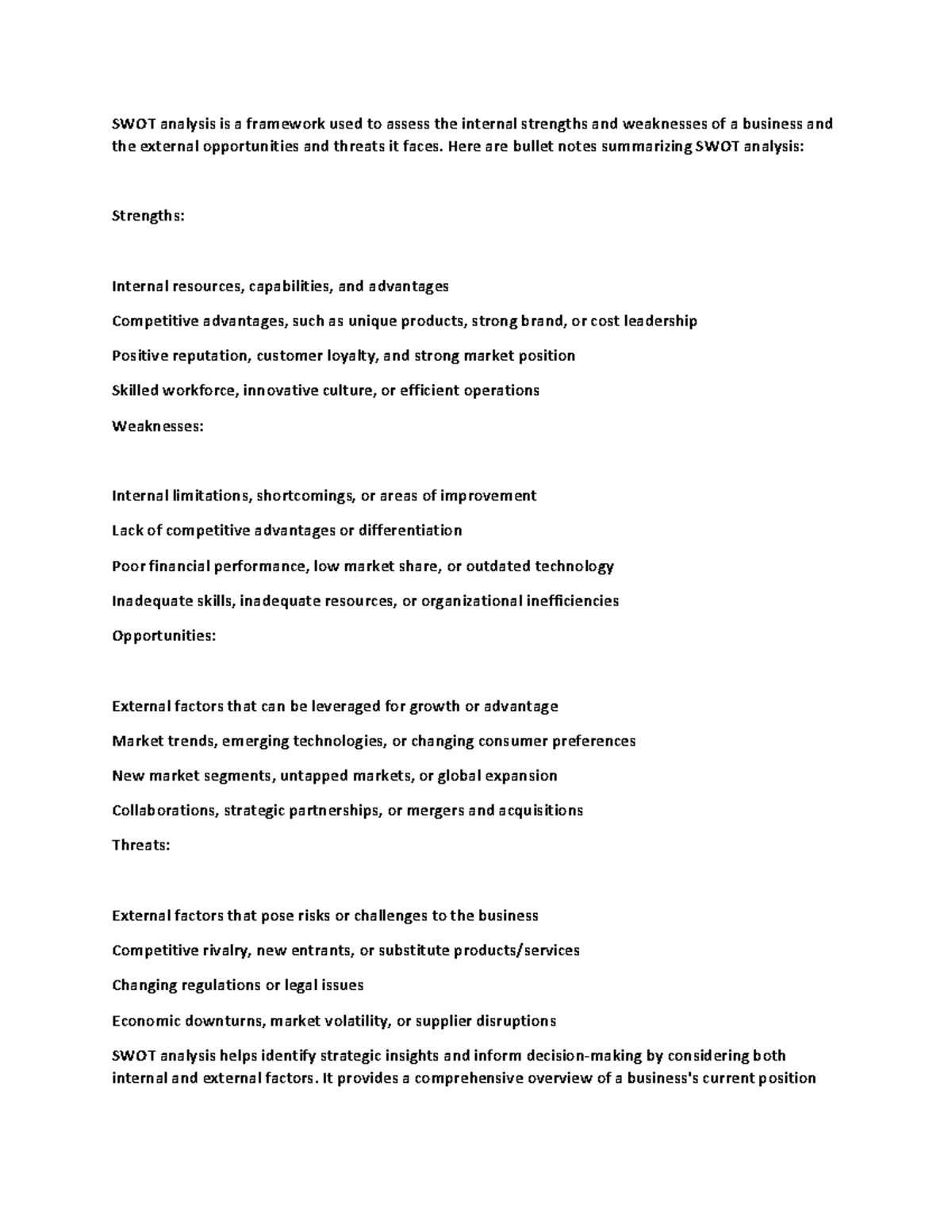**Caption:**

This image displays a printout detailing a SWOT analysis, a strategic framework used to evaluate a business's internal strengths and weaknesses, alongside external opportunities and threats. 

At the top, the text elaborates on the purpose of SWOT analysis, emphasizing its role in assessing both internal and external factors affecting a business. 

The strengths section outlines key internal resources such as unique products, strong brand or cost leadership, positive reputation, customer loyalty, and skilled workforce. It also highlights competitive advantages like an innovative culture or efficient operations.

The weaknesses section identifies internal limitations and areas of improvement, including lack of differentiation, poor financial performance, low market share, outdated technology, inadequate skills, resources, or organizational inefficiencies.

In the opportunities paragraph, the text describes external factors that could drive growth. These include market trends, emerging technologies, changing consumer preferences, new market segments, untapped markets, global expansion potential, strategic partnerships, and mergers and acquisitions.

The last paragraph focuses on threats, though its detailed content is not visible in the image. This structured analysis serves as a comprehensive guide for understanding the various factors influencing a business’s strategic planning.